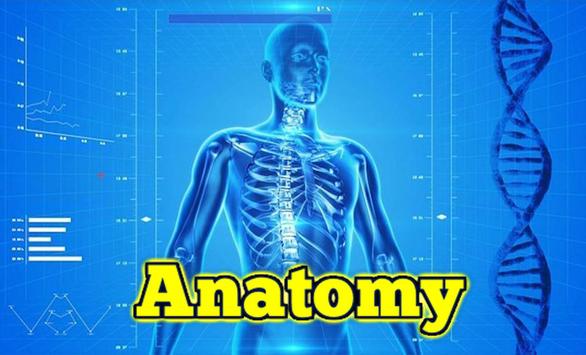This image is a highly stylized and anatomically accurate blue illustration of a human figure that has a robotic appearance. The figure is centrally placed and semi-transparent, revealing the skeleton with visible spine, ribcage, and some bones in the arms underneath the chest area. The background is predominantly blue, transitioning from darker shades on the edges to lighter tones towards the center. On the right side of the image, there is a dark blue rendering of a DNA helix, while the left side features technical charts and graphs on white relief. At the bottom of the image, large yellow lettering with a black outline spells out "ANATOMY" in front of the human figure, set against the monochromatic blue background. The overall color scheme, aside from the white elements, is various shades of blue.